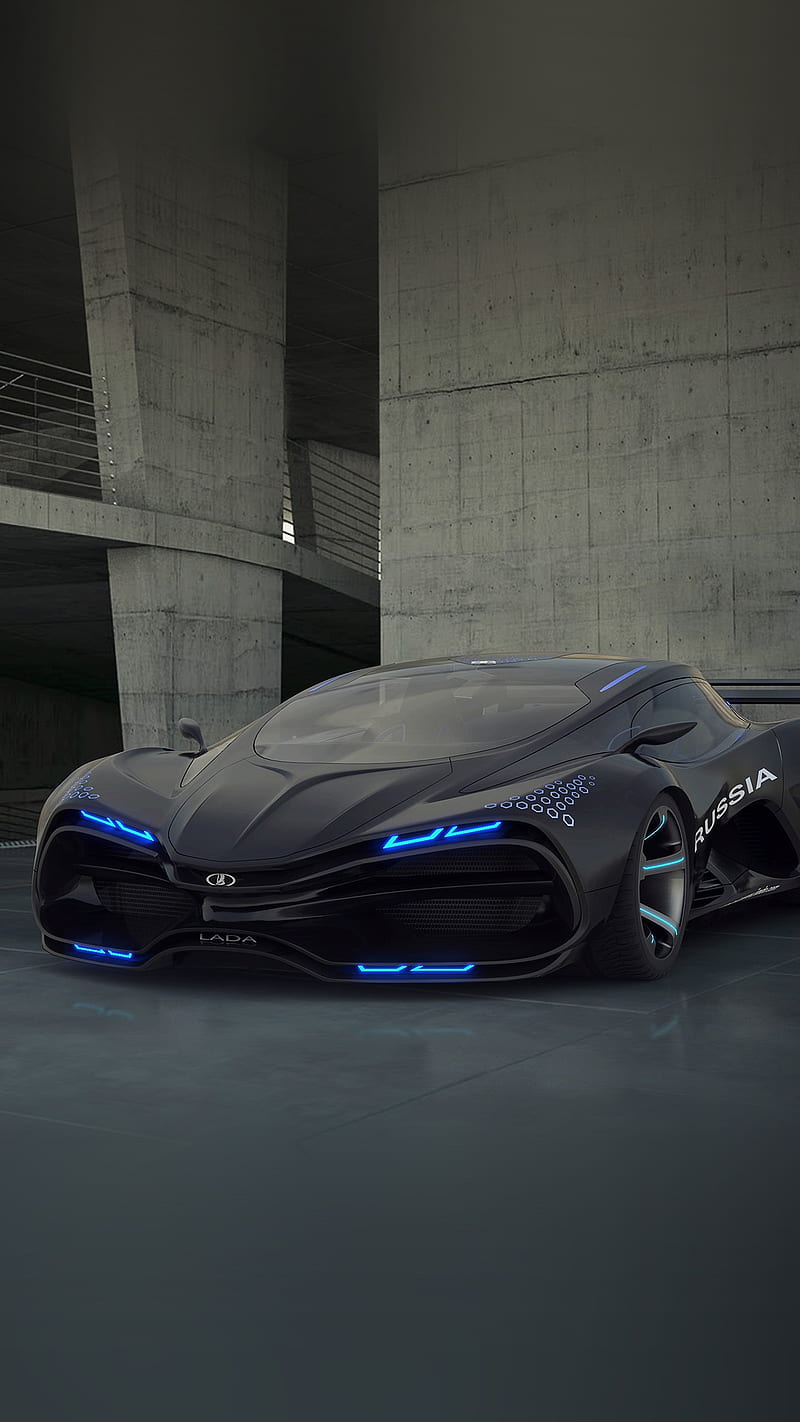The image showcases a super sleek, black sports vehicle reminiscent of a Batmobile, parked in a stark, brutalist-style concrete warehouse or parking garage. The vehicle's ground-hugging, streamlined body features an undulating, Stingray-like silhouette, accentuated by vivid blue headlights and similarly hued lights on the hubcaps of the visible front left tire. The frontal design includes a distinctive hourglass shape with headlights and a central emblem that resembles a circle with detailing, plus text reading "LADA." Intriguingly, the driver's side door is marked with the word "Russia." The car's modern, futuristic design is emphasized by its curved, sunroof-like front window, giving it an almost digitalized appearance. The surrounding environment is industrial, with gray concrete pillars and walls, and visible wiring near one of the pillars, all contributing to a raw, edgy setting.